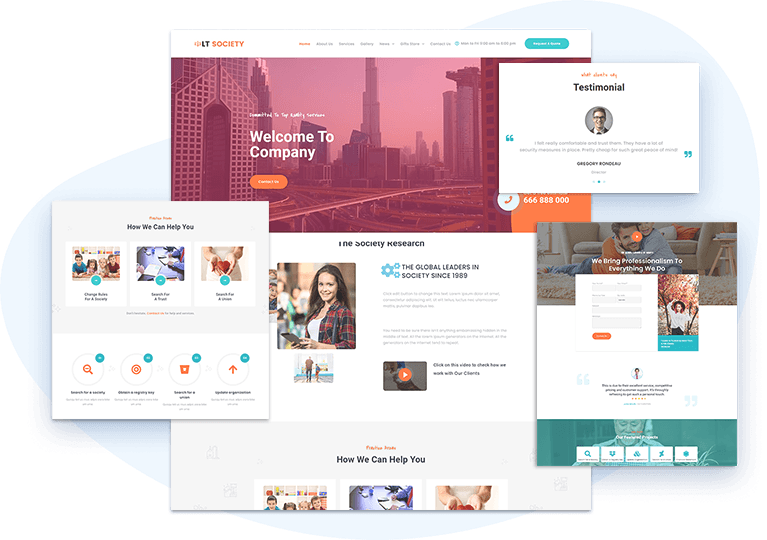This image captures the homepage of a website, featuring various elements and pop-ups. The overall backdrop is white complemented by blue bubbles. The central image, the largest one in the background, is displayed in portrait orientation with a predominantly white background. At the top, it prominently features the text "LT to Society" where "LT" is in black and "Society" in orange. Below this header, there is a navigation bar with several options that are too small to decipher.

A prominent green oval-shaped button with white text is included, though the specific wording is unclear. Beneath this, a red landscape background overlays a transparent cityscape with white text stating "Welcome to the Company." Further down, there's an image titled "The Society Researcher," showcasing a photo of a woman alongside the phrase "Global Leaders in Society Since 1989."

To the left, there is a pop-up box saying "How Can We Help You?" featuring three icons within blue circles, accompanied by additional white and orange icons below. Another pop-up on the left displays a man being hugged by a child, along with input fields for entering personal information and signing up.

Above this pop-up, a rectangular white box with orange font displays the word "Testimonial," followed by black text and the avatar of a man wearing glasses and a suit. His testimonial is partially visible, and his name appears to be Gregory, though the last name is not legible.